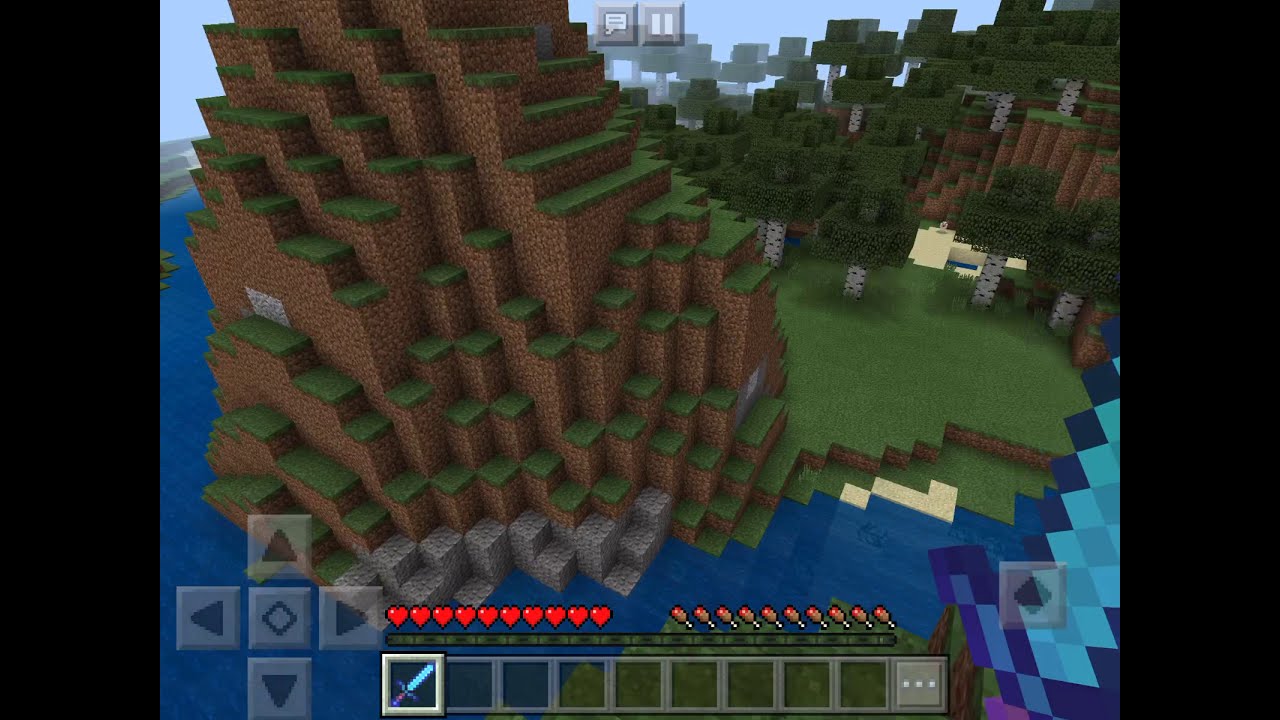This image depicts a first-person view from a Minecraft game, showing a player holding a detailed blue sword with a dark blue hilt, purple handle, and lighter blue blade, with a full health bar and additional menu icons at the bottom. The scene is flanked by vertical black letterbox bars on either side, intensifying focus on the central landscape. The central mountain structure is highly intricate, resembling an Escher-like stair-step pattern. It features layers of brown dirt and green grass atop each step, descending to a gray, rocky base that blends into dark blue water on one side and transitions into grassy land on the other. This land connects to a forest with towering pine trees, which ascend another mountain in the background. The expansive view includes a mix of additional green and brown terrain, suggesting a continuous, sprawling Minecraft world with an ocean visible further in the distance.